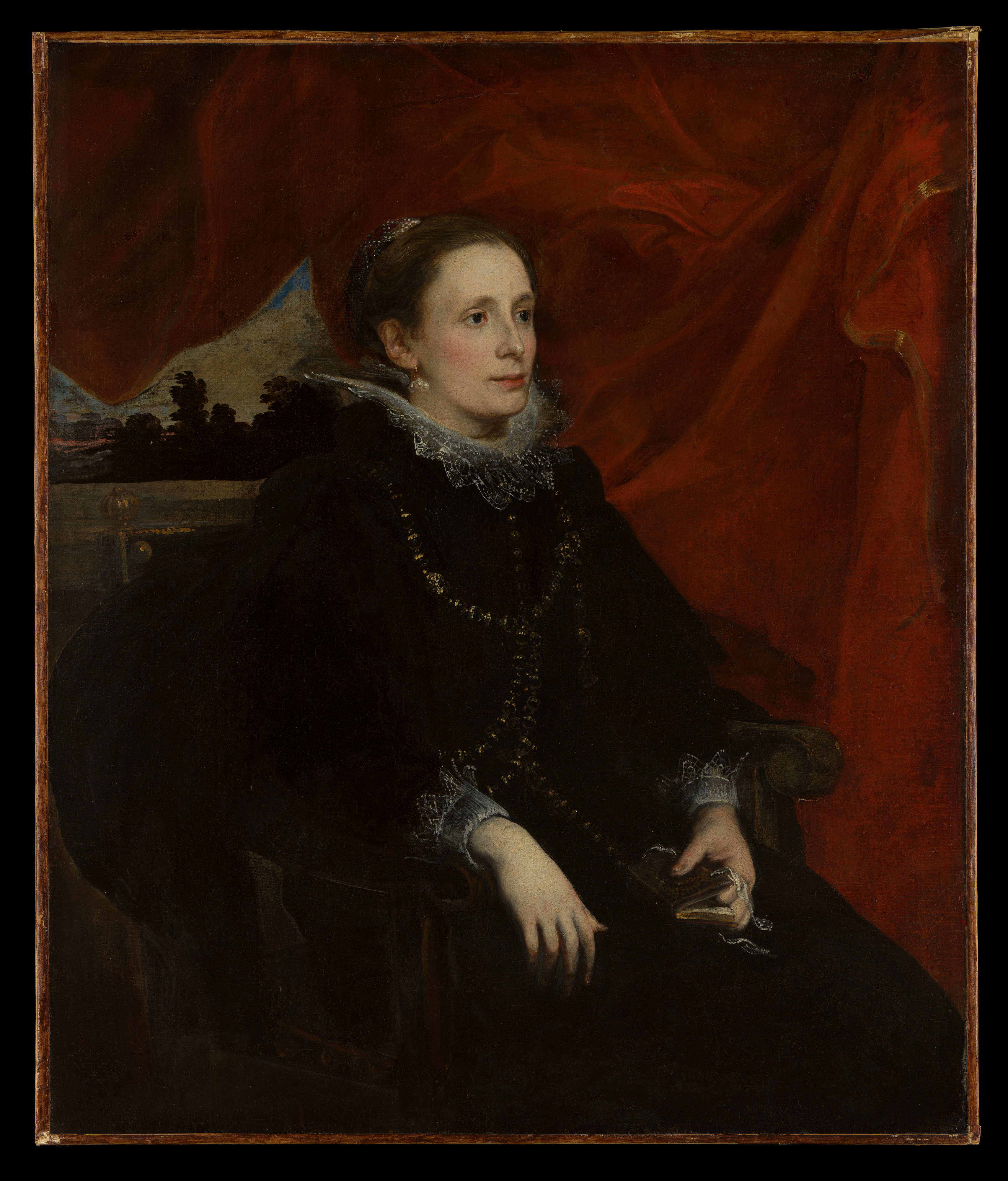The portrait showcases a young Caucasian woman dressed in a Victorian-era satin black dress adorned with intricate light gray lacework detailing around the broad collar and cuffs, and accented with light golden accessories. Her hair is neatly styled in a bun at the back of her head, and she is wearing earrings, pink blush, and red lipstick. The woman's posture is relaxed, sitting in a wooden chair with her elbows resting on the armrests and her hands placed on her lap, holding a small brown bound pocketbook. She is positioned in a three-quarter profile, facing forward and to the right, causing her gaze to be directed around the 3:30 position. 

The background features a dark red, loosely wrinkled cloth, creating a rich, textured backdrop. The portrait appears to be quite dimly lit, with her face and hands standing out in bright contrast against the darker tones. Additionally, there is a hint of a scenic landscape in the very distant background, including what might be snow-covered mountains and green trees or bushes. The edges of the portrait are bordered by a thin golden line, mounted within a dark brown frame, enhancing the classical and timeless quality of the painting.